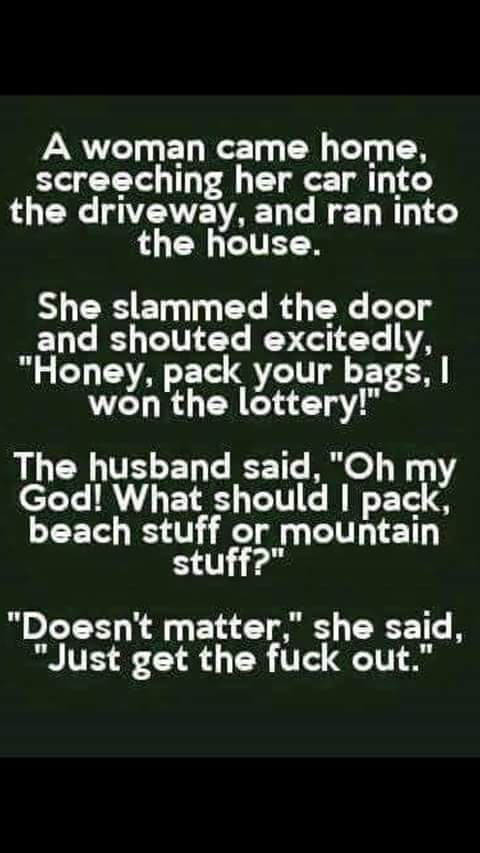The image depicts a joke in white letters on a black background. It reads: "A woman came home, screeching her car into the driveway, and ran into the house. She slammed the door and shouted excitedly, 'Honey, pack your bags! I won the lottery!' The husband said, 'Oh my god, what should I pack—beach stuff or mountain stuff?' She replied, 'Doesn't matter, just get the fuck out.'" The text includes appropriate punctuation, quotes, and capitalization, emphasizing the humorous exchange between the couple.